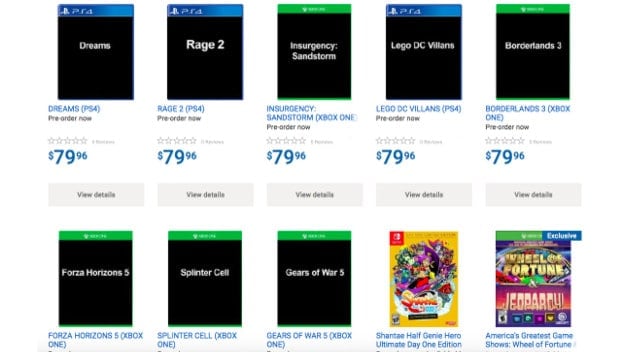In this image, a lineup of video game boxes is showcased, organized predominantly by console type and title. At the top, five black boxes for the PlayStation 4 and Xbox One games are displayed. Starting from the left:
1. A PS4 game titled "Dreams," encased in a black box with white font, priced at $79.96 in blue.
2. Next, "Rage 2" for the PS4, featuring a black background with white lettering, also marked at $79.96.
3. The third box is "Insurgency: Sandstorm" for Xbox One, labeled with a "Pre-order Now" tag, priced similarly at $79.96.
4. Followed by "Lego DC Villains" for PS4, again tagged at $79.96.
5. Lastly, "Borderlands 3" for Xbox One, maintaining the same price of $79.96.

Below these, in a segment encouraging viewers to explore further deals, a line of gaming titles from various genres and platforms is listed in gray-black font. From left to right:
1. "View Deals" featuring "Forza Horizon 5" for Xbox One.
2. "Tom Clancy's Splinter Cell" for Xbox One.
3. "Gears of War 5" for Xbox One.
4. "Shantae: Half-Genie Hero Ultimate Day One Edition," presented with a vibrant orange background adorned with central imagery.
5. "America's Greatest Game Shows: Wheel of Fortune & Jeopardy" with the "Wheel of Fortune" title highlighted in gold, and "Jeopardy" in pink against a reddish backdrop.

This curated selection not only showcases popular gaming titles but also promotes ongoing deals, encouraging enthusiasts to dive into a variety of gaming experiences across different consoles.